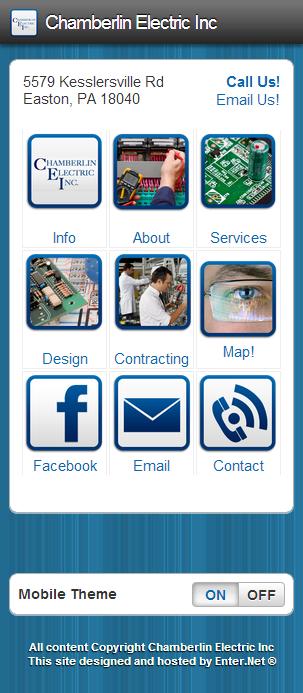The image is a screenshot of a smartphone displaying an outdated and basic-formatted website for Chamberlain Electric Inc., which is located at 5579 Kesslersville Road, Easton, PA, 18040. At the top, there is a black banner with white text that reads "Chamberlain Electric Inc." Below it, a blue banner with a white rectangle contains multiple sections. In the top left corner, the address is written in black text, while "Call Us" and "Email Us" appear in blue text on the top right. The website includes several icons and text categories arranged in three rows: Info, About, Services, Design, Contracting, Map, Facebook, Email, and Contact. At the bottom, a bluish-gray bar with a white section offers a toggle for the 'Mobile Theme', with the option switched on. The very bottom of the screen states, "All Content, Copyright, Chamberlain Electric Inc. This site designed and hosted by Enter.net."